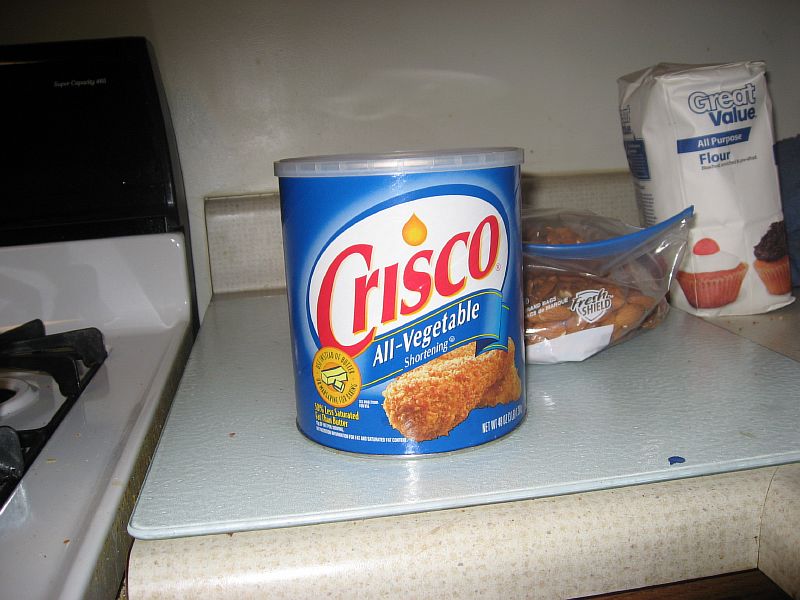The image depicts a cluttered kitchen countertop with various items, focusing predominantly on a large, blue can of Crisco all-vegetable shortening. The can, which features a white oval with 'Crisco' written in red, displays an image of golden-brown fried chicken, emphasizing its crusty, buttery flavor ideal for cooking. This Crisco can, with a white plastic top, sits centrally on the countertop. Behind it, on the right, is a transparent zip-lock bag containing what appears to be cookies. Further to the right is a five-pound bag of Great Value all-purpose flour, which is white with an image of two cupcakes on the label. The countertop is white and slightly dirty, paralleling the condition of the white gas stove visible to the left. The stove, which has black details, appears somewhat stained with specks of yellow and orange food residue, indicating recent usage. The wall behind the counter is also white, contributing to the overall untidy yet homey kitchen scene.